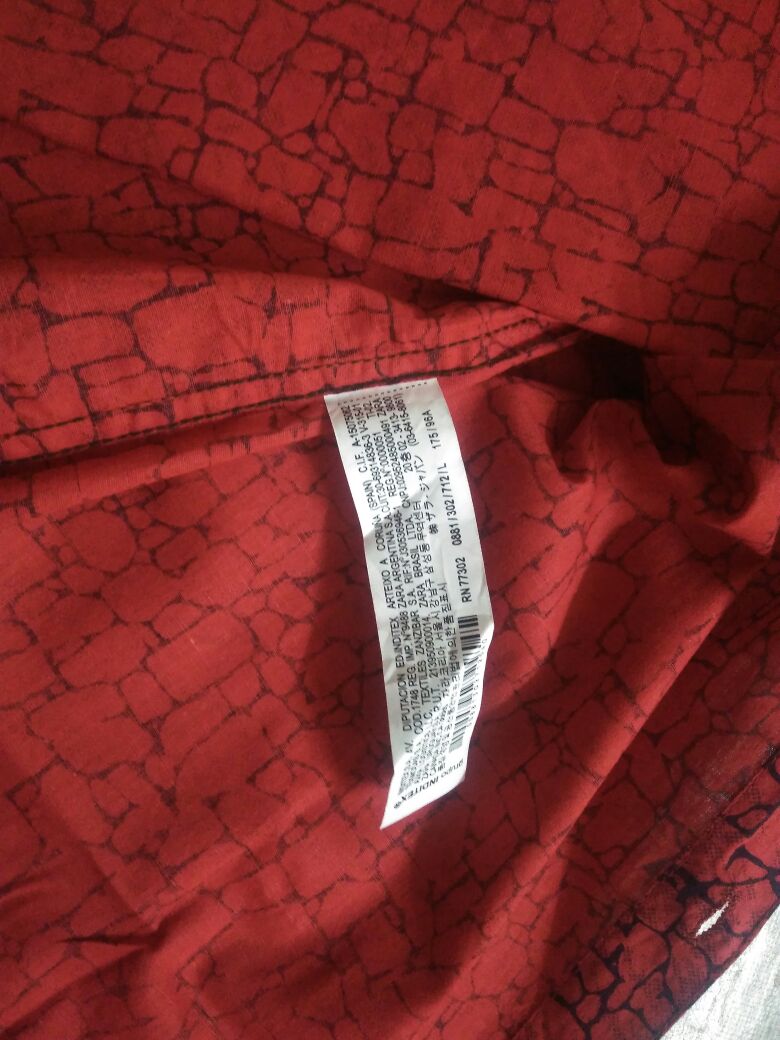The image showcases a vividly detailed close-up of a piece of fabric, likely the inside of an article of clothing, possibly a shirt or a pillowcase. The fabric is predominantly magenta red with a maroon tint, covered in an intricate pattern of interlocking black outlines that resemble medieval cobblestone walls or cracked dirt. These shapes—squares and rectangles of various sizes—create a visually cohesive and somewhat textured design. In the center of the image is a vertically-oriented, long rectangular white tag with small black print that is difficult to decipher, suspended from one of the seams. The tag appears to be composed of a satiny material and contains care instructions in multiple languages, including Spanish and Chinese, as well as various numbers and a barcode. The brand name "Zara Brazil" is visible, indicated that the item may be made for the Brazilian market. The bottom right corner reveals a seam and a single buttonhole, hinting that the item can be fastened securely.